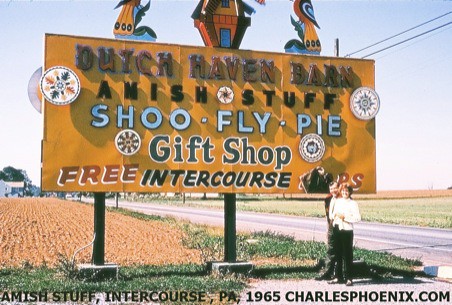In the bright, postcard-perfect photograph, a cheerful couple stands beside a roadside attraction sign, both smiling warmly at the camera. The woman, radiant in white, and the man, dapper in a dark suit, create a charming contrast against the sunny outdoor setting. The sign, which is rectangular and vibrantly orange, features a mix of stylized Indian and Amish motifs. It proudly advertises "Dutch Haven Barn," "Amish Stuff," "Shoe Fly Pie," "Gift Shop," and intriguingly, "Free Intercourse." The bottom of the sign further reads "Amish Stuff, Intercourse, PA, 1965, CharlesPhoenix.com." All of this is set along a tranquil country road that meanders into the distance, flanked by sprawling farm fields and a patch of green grass, epitomizing rustic charm.